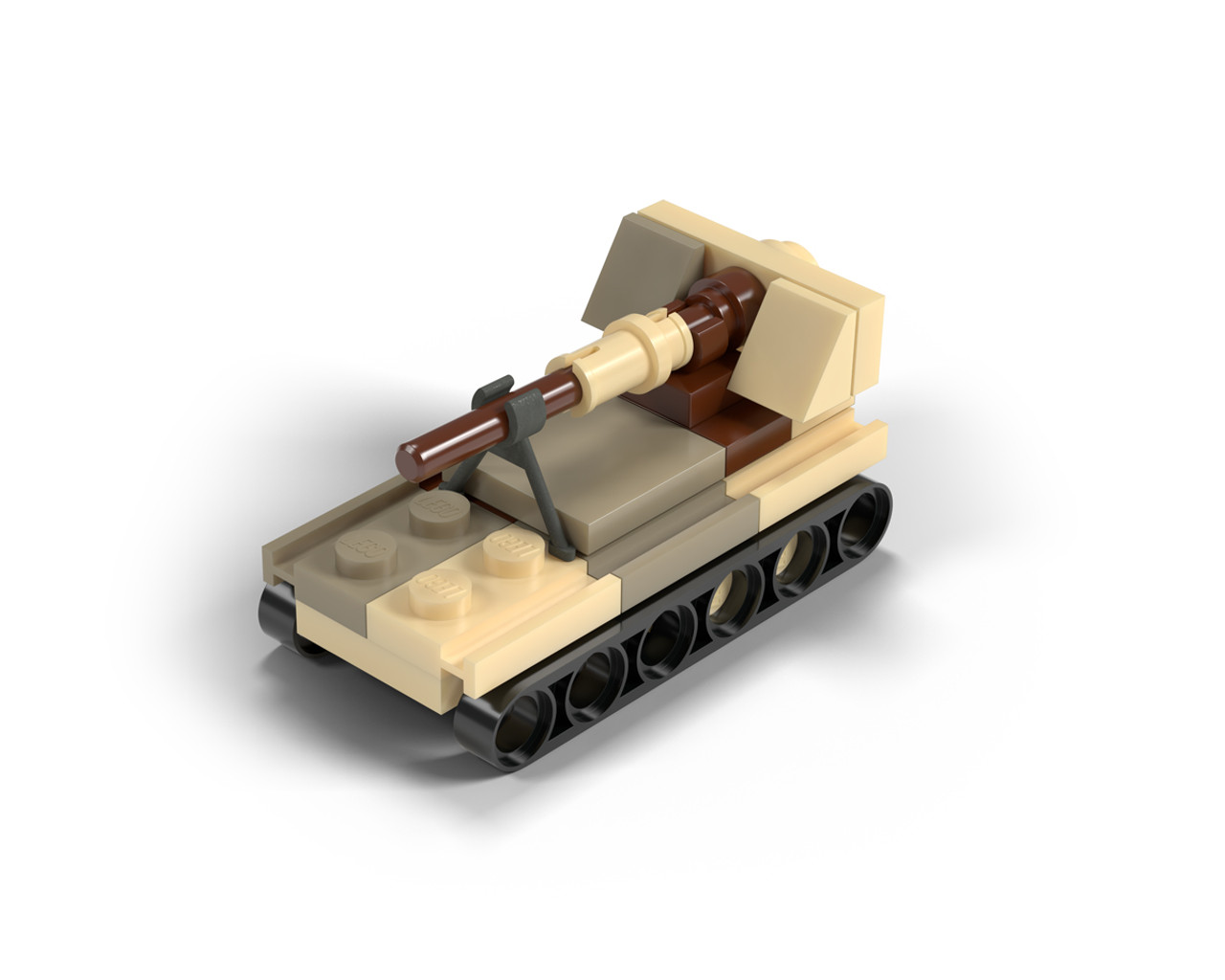The image depicts a small, custom-designed LEGO tank, meticulously assembled. The tank features a black base with distinct black treaded wheels. The body of the tank is constructed using a mix of white, light tan, and gray LEGO blocks, providing a contrasting yet cohesive color scheme. Notably, the tank's gun barrel is a slim, dark cherry brown cylinder supported by a gray stand. The assembly appears intentional and detailed, rather than makeshift, showcasing a compact design with about 12 to 15 LEGO pieces. Despite its simplistic appearance, the design clearly resembles a tank, complete with a realistic tread mechanism and a well-defined turret.